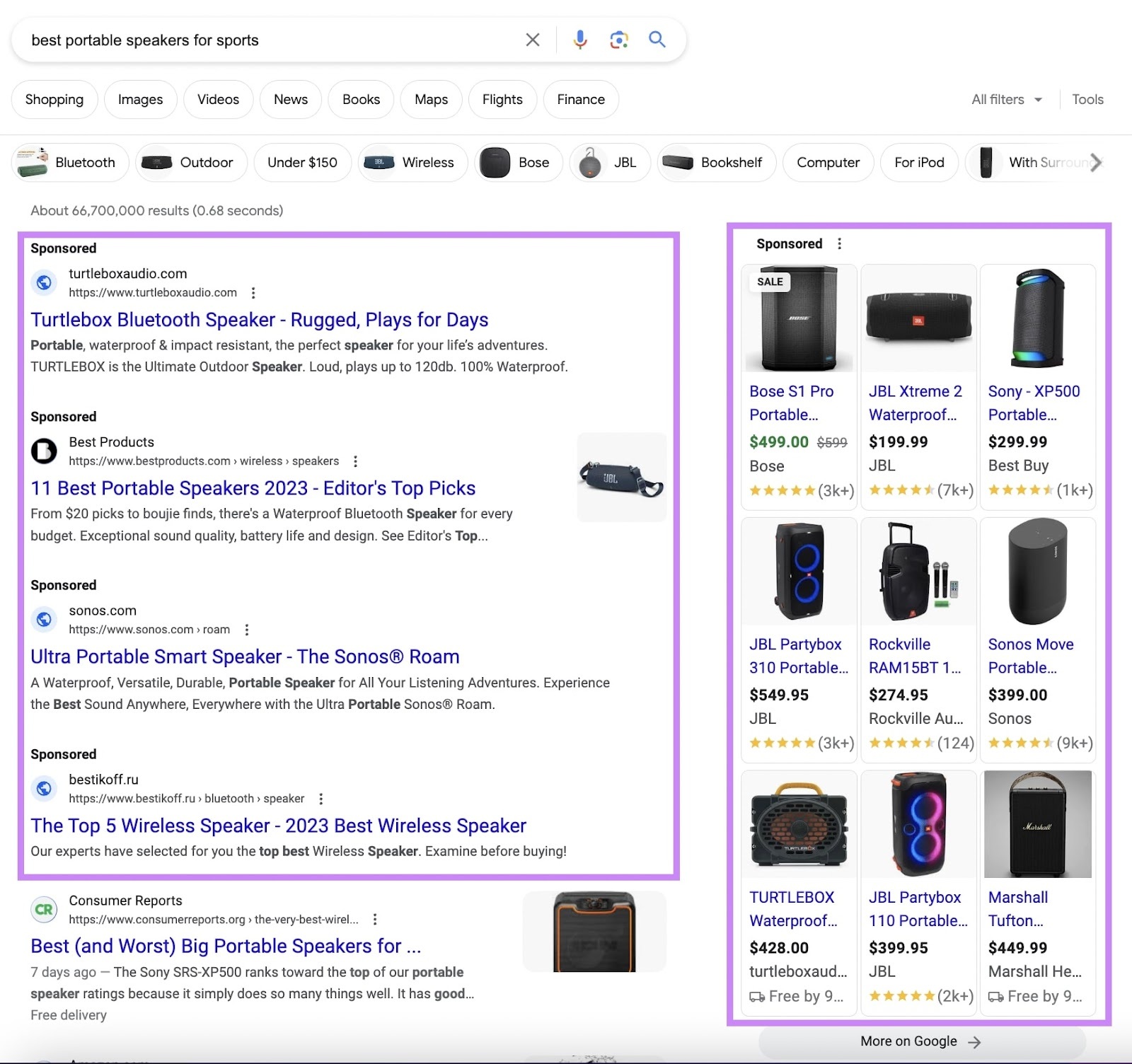This image is a detailed screenshot of a Google search for "best portable speakers for sports." The search box, located in the top left corner, features Google's signature color scheme with emblems for voice search (microphone), photo search, and regular search (magnifying glass). Below the search box, a row of white buttons provides options to filter results by Shopping, Images, Videos, News, Books, Maps, Flights, and Finance. Additionally, there are drop-down menus on the right for "All filters" and "Tools."

Directly beneath these filters, there are white suggested search buttons, arranged from left to right, labeled: Bluetooth, outdoor, under $150, wireless, Bose, JBL, bookshelf, computer, for iPod. Some of these labels are cut off, followed by an arrow indicating the availability of more suggestions.

The search has yielded approximately 66,700,000 results, generated in 0.68 seconds. Featured prominently, a purple box encircles the top four results, identifying them as sponsored search results. Below these sponsored results, the first non-sponsored result is from Consumer Reports, situated at the bottom of the page.

On the right-hand side, occupying about one-third of the page, another purple box highlights nine images of various portable speakers. These images include vital details such as pricing, reviews, and ratings, and are part of the sponsored ads section.